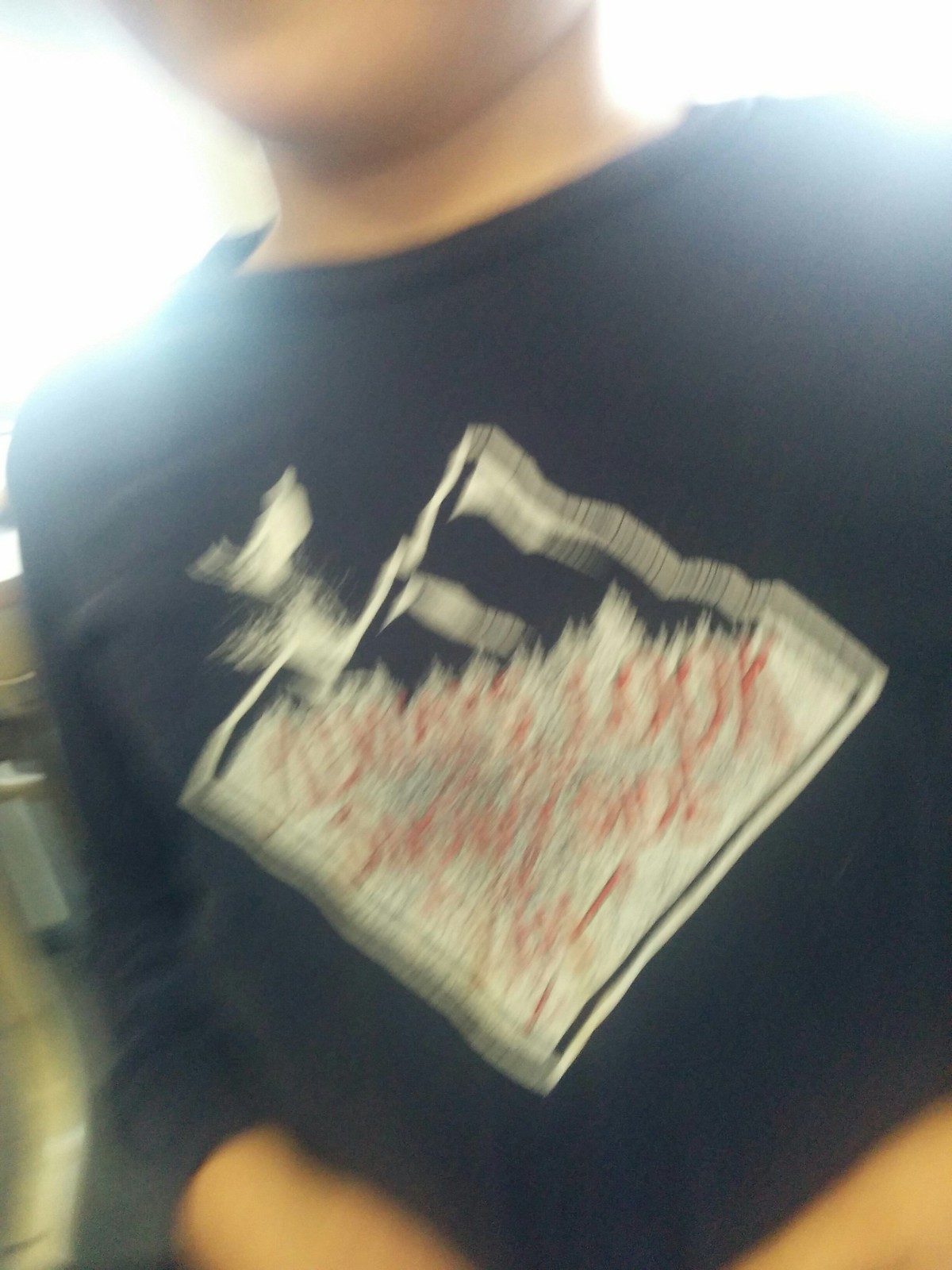A close-up, blurry photograph shows a person, likely male, from the chin to the waist. The individual is wearing a blue long-sleeve t-shirt. Only parts of his hands are visible at the bottom of the frame, seemingly resting on his lap. The front of the shirt features a large, intricate design resembling a diamond shape. Within the diamond, there's an illustration of white pine trees along with what seems to be red, scribbly stripes underneath. Due to the blur, other parts of the design appear indistinct and blotchy.